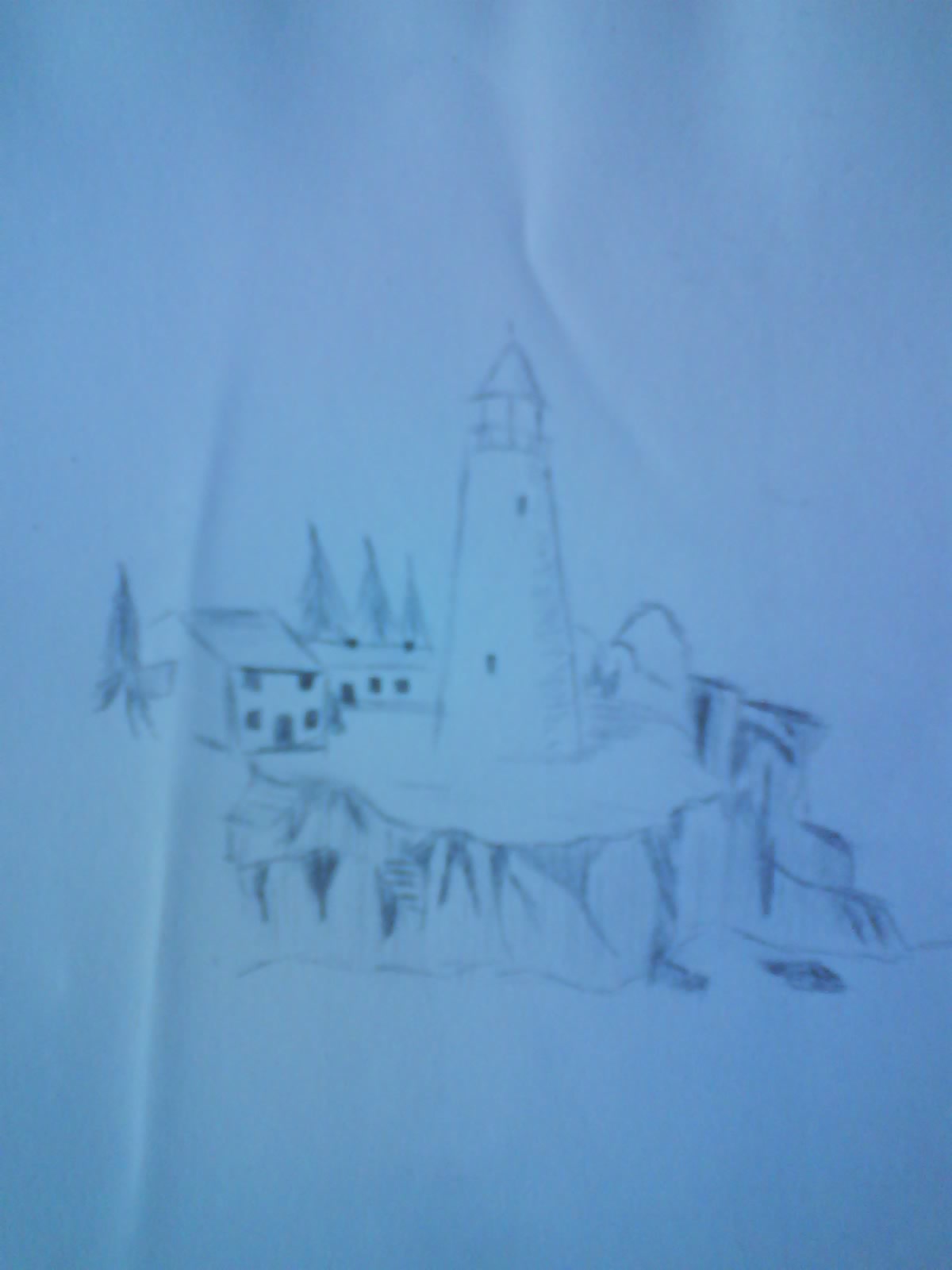This image is a somewhat blurred photograph of a hand-drawn pencil sketch on slightly wrinkled white paper, giving it a washed-out, blueish appearance. The central focus of the drawing is a lighthouse that stands on the edge of a rocky cliff. The lighthouse, a tall, tapered tower, features staggered windows—one lower on the left and one higher on the right. Just below the tower's pointed cap roof is a railed balcony, encircling the glass windows where light would typically shine out. 

At the base of the lighthouse on the right, there is a flat, circular area surrounded by a wall. Adjacent to the lighthouse on the left, two smaller buildings are drawn; one is a two-story house with a door and four windows, while the other has a door and two windows. Additional details include several trees scattered around the area. The overall scene, rendered in shades of gray, combines elements of both a rocky maritime setting and a fortified castle-like structure, highlighted by its slightly ethereal, blue-toned photograph.